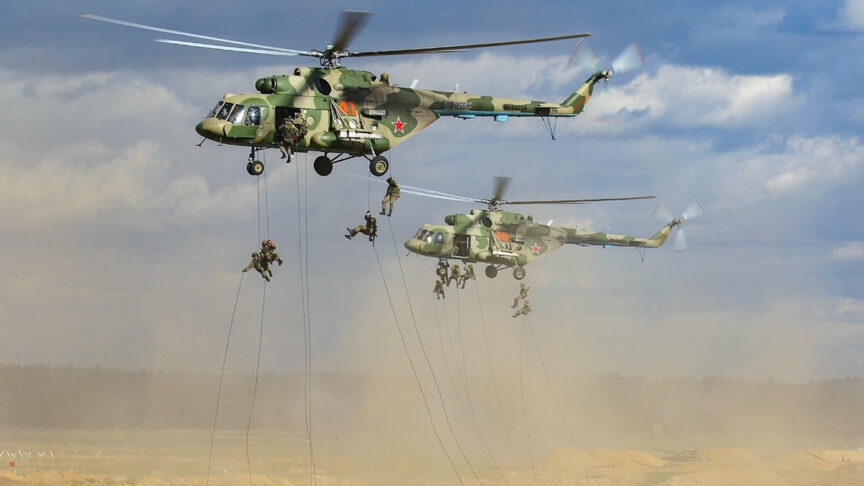In this dynamic action photograph, two military helicopters, adorned with a blended camouflage pattern of green and brown and marked by red stars on their tails, hover over a sandy desert landscape. The sky above is a clear blue punctuated by fluffy white clouds, with distant hills or mountains faintly visible in the background. The powerful motion of the helicopters' propellers stirs up plumes of dust, adding a brown haze to the scene. Suspended by ropes, approximately 14 soldiers dressed in green camouflage uniforms are rappelling down—four to five from the leading helicopter on the left and about 10 from the one slightly behind it on the right. The image captures a vivid moment of a military operation or drill, emphasizing the precision and coordination of the personnel amidst the harsh, sandy environment.